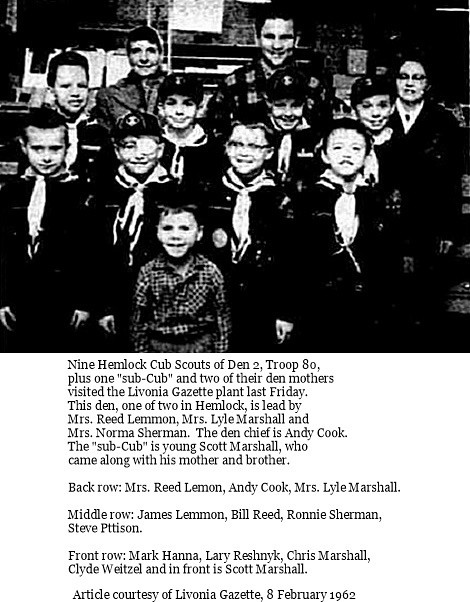The black and white photograph captures a nostalgic scene from February 8, 1962, featuring a group of twelve individuals—two adults and ten boys—dressed predominantly in Boy Scouts or Cub Scouts uniforms. The scouts are arranged in three rows, with the adults standing in the back. The image is slightly blurred, and the details are somewhat hard to discern due to its age and quality. Nonetheless, the uniforms are distinguished by neckerchiefs, and the boys display joyful expressions, except for a very small child at the front dressed in a checkered shirt.

The accompanying text below the image introduces the group as nine Hemlock Cub Scouts of Den 2, Troop 80, along with one "sub-Cub" and two of their den mothers who visited the Livonia Gazette plant. Den 2, one of two dens in Hemlock, is led by Mrs. Reed Lemon, Mrs. Lyle Marshall, and Mrs. Norma Sherman. The Den Chief is Andy Cook, and the sub-Cub is young Scott Marshall, who is present with his mother and brother.

In the back row, from left to right, stand Mrs. Reed Lemon, Andy Cook, and Mrs. Lyle Marshall. The middle row includes James Lemon, Bill Reed, Ronnie Sherman, and Steve Tissen. The front row features Mark Hamma, Larry Reschnick, Chris Marshall, Clyde Wetzel, and, positioned at the very front, little Scott Marshall. This charming historical snapshot is documented in Article 33 of the Livonia Gazette, dated February 8, 1962.